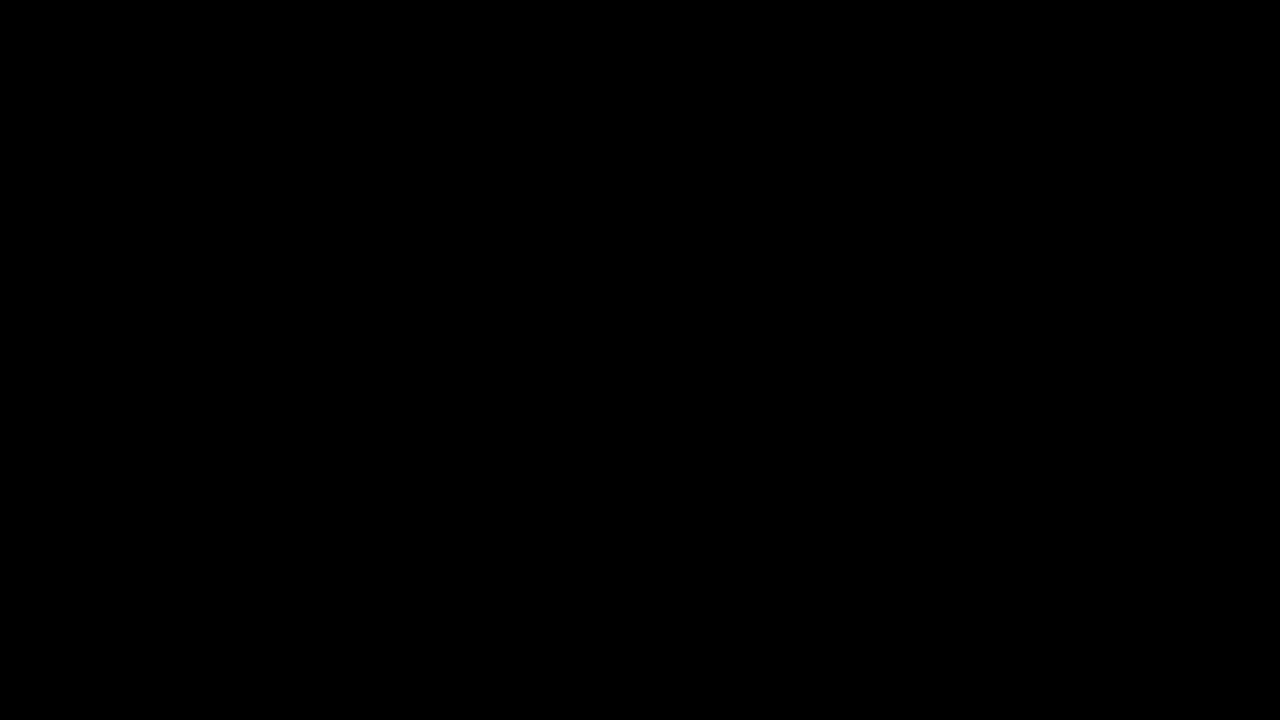The image is a solid black rectangle, with a width approximately twice its height, measuring roughly 8 inches wide by 6 inches high. Every pixel within the image is uniform and dark black, without any hint of variation or discernible features. The corners are precisely 90 degrees, and the edges are perfectly straight, resulting in a flawless rectangular shape. Despite close inspection for any subtle shades, patterns, or signs of life, the image remains consistently and entirely black, akin to the emptiness of a void or a blank chalkboard.